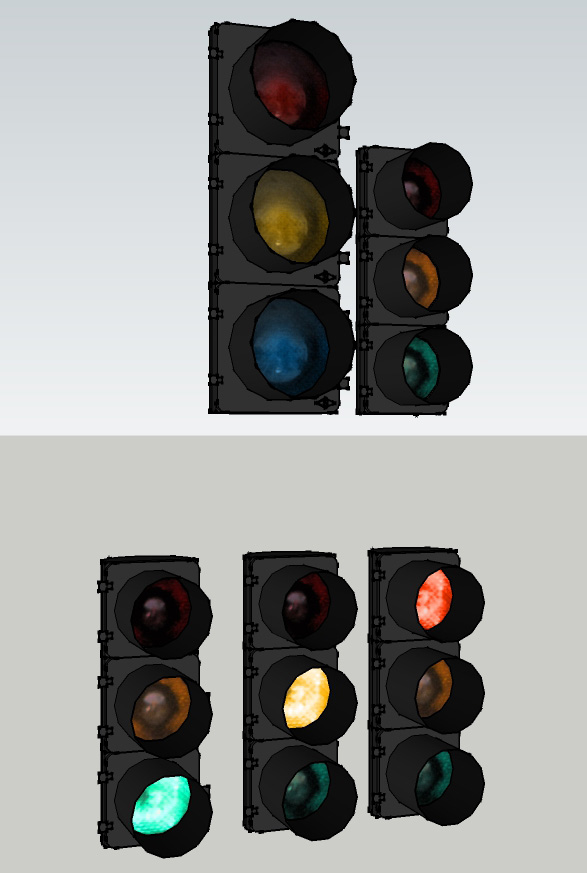The image is a composite of two illustrations featuring traffic lights set against different colored backgrounds. The upper section displays two traffic lights on a blue backdrop. The traffic light on the left is uniquely colored with red, yellow, and blue lights, while the one to its right features the standard red, orange, and green lights. Notably, none of the lights in the upper image are illuminated. In the lower section, there are three traffic lights on a gray background, each with a black structure. From left to right, the traffic lights are traditionally colored with red, orange, and green lights, but each displays a different active light: the leftmost traffic light has the green light illuminated, the middle one shows the yellow light, and the rightmost light has the red light lit. All these lights appear to be of the same size in the lower image.